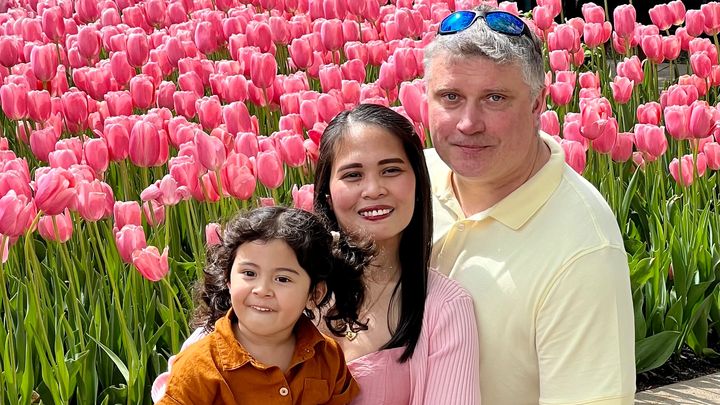In this vibrant, outdoor close-up photograph, a family of three is captured standing in front of a striking backdrop of blooming pink tulips. At the center of the image, a young girl with pigtails and curly brown hair is beaming, showing her teeth. She is wearing a tan shirt and appears to be Indian or Hispanic. Hugging her from behind is a woman presumed to be her mother, with long brown hair and tan skin, smiling warmly in a pink shirt. To their left stands a man, likely the father, with short salt-and-pepper hair, wearing a yellow polo shirt and sunglasses perched on his head. His light-colored eyes are fixed on the camera, and he too is smiling. The background is densely packed with layers of pink tulips, creating a lush and colorful setting. A small path or sidewalk is visible in the lower right-hand corner, adding a subtle detail to the lively floral scene.